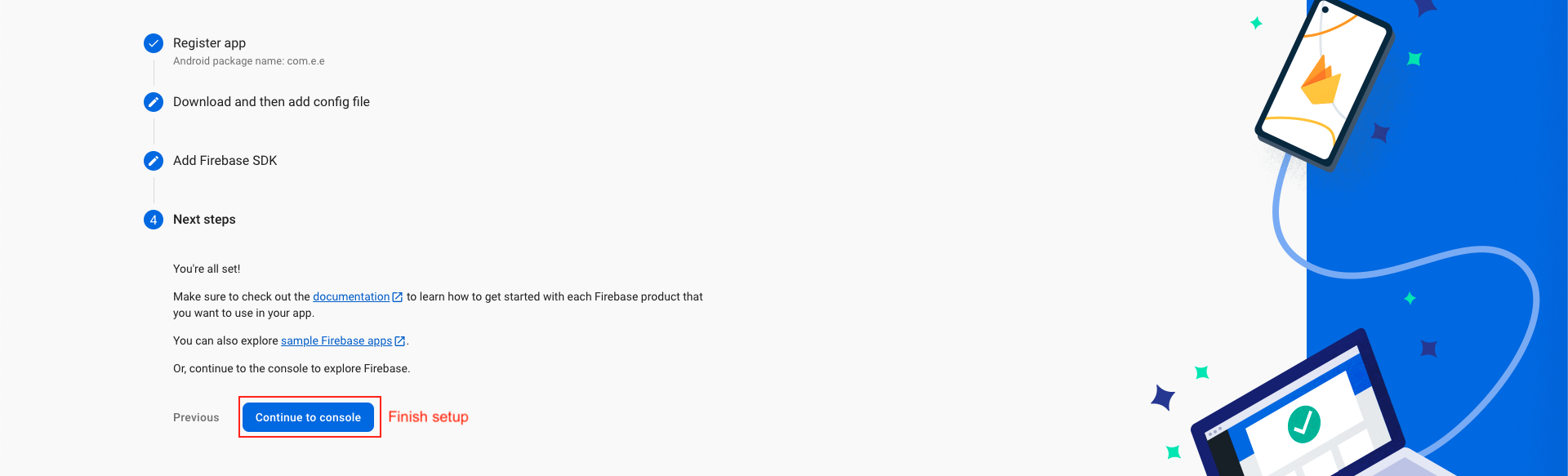This is a detailed screenshot of an app installation page, presented in a wide rectangular format and oriented horizontally on the screen. The right half of the rectangle features a blue background that runs vertically down the screen. At the top of this blue section, there is an image of a smartphone positioned diagonally, pointing towards the upper right corner. A blue line, shaped like an S, winds its way down from the smartphone to the bottom of the page, where it culminates in an illustration of an open laptop, which is tilted diagonally to the left. 

Surrounding the smartphone and laptop are multicolored star shapes in shades of blue and green, adding a decorative touch. 

The left side of the page is dedicated to a series of instructional steps for setting up the app. These steps include:
1. Register the app.
2. Download.
3. Add config file.
4. Add Firebase SDK.
5. Next steps.

At the bottom left of the page, there is a prominent blue rectangle with the text "Continue to Console" centered within it, inviting the user to proceed.